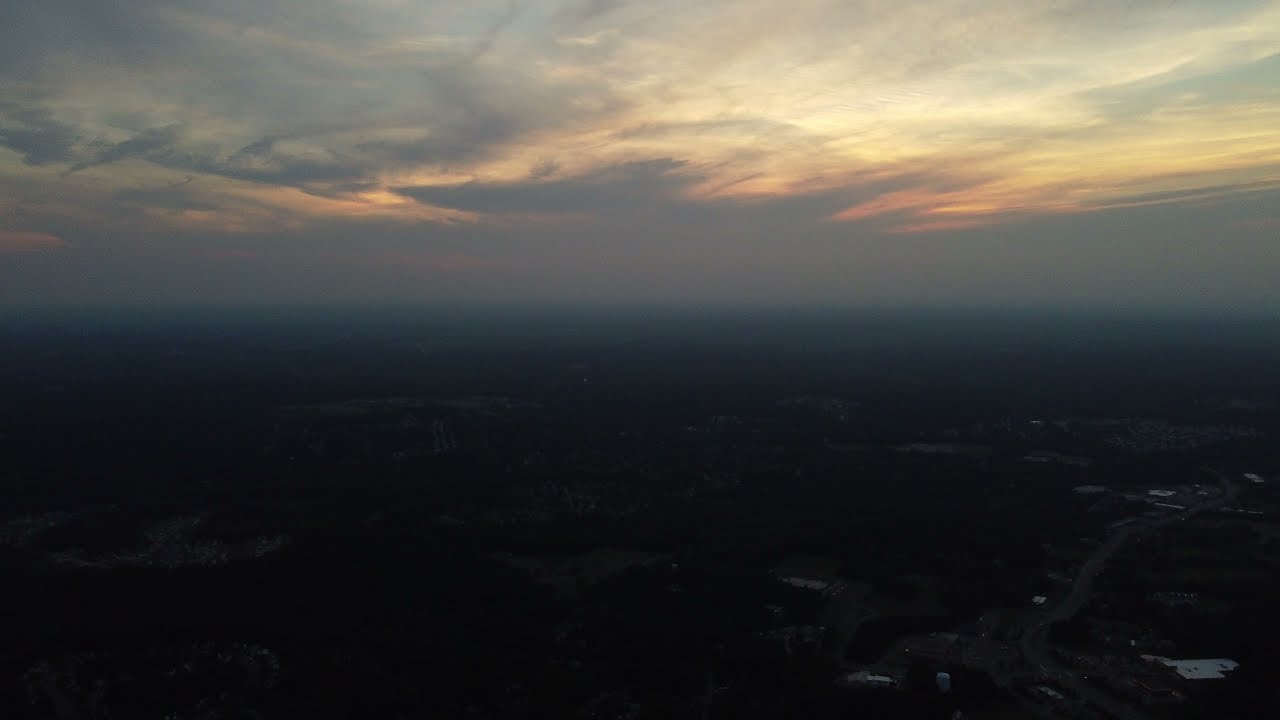This photograph, seemingly taken from an airplane at a high altitude, offers a sweeping view of the land below and the sky above. The image is somewhat blurry and grainy, indicative of a spontaneous capture, possibly to commemorate a journey. The upper half of the photo features a dramatic sky, with white clouds partially obscuring a setting sun. Rays of reddish, orangish, and yellow-gold light pierce through the clouds, casting a beautiful gradient that transitions into a blue sky. The lower half is shrouded in darkness, with faint glimpses of land, roads, trees, small bodies of water, and a scattering of buildings. Despite the lack of sharp detail, the contrast between the vibrant sky and the shadowy terrain creates a visually striking scene that holds sentimental value for the photographer.